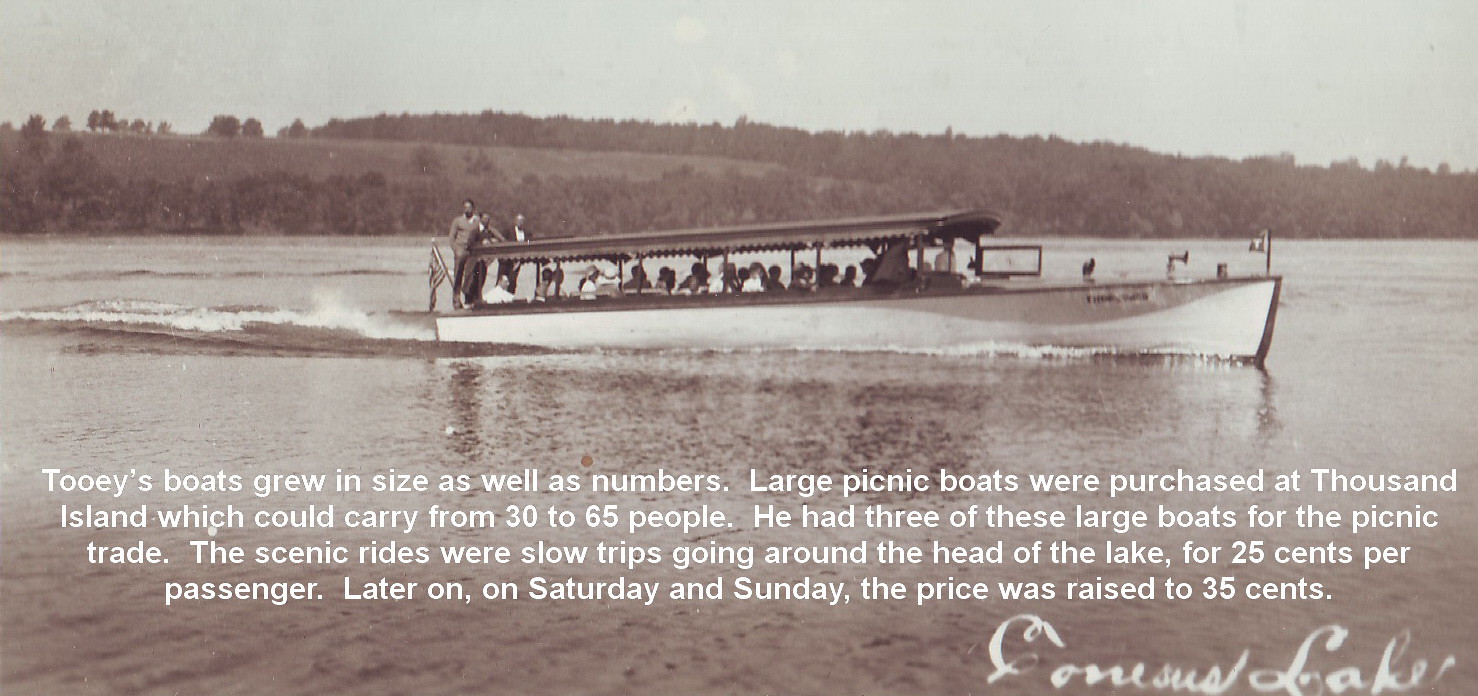This black-and-white photograph, approximately six inches wide and three inches tall, captures a serene daytime scene at Conesus Lake. The lower portion of the image is dominated by the water, with the upper section showcasing low-lying hills dotted with trees beneath an open sky, indicating a season outside of winter or late fall. Central to the composition is a large picnic boat, approximately 50 feet long, adorned with a canvas canopy under which numerous passengers are seated. At the boat's bow, exhaust pipes and a brass bell are visible, while at the stern, three men stand beside an American flag and the motor. The boat, part of Tuohy's fleet, ferried 30 to 65 people on leisurely scenic rides around the lake for a fare of 25 cents per passenger, later increased to 35 cents on weekends. The photograph's historical context is further detailed in white text below the image, explaining the evolution and expansion of Tuohy's boats, and in the lower right-hand corner, "Conesus Lake" is inscribed in white cursive, anchoring the photograph's location.